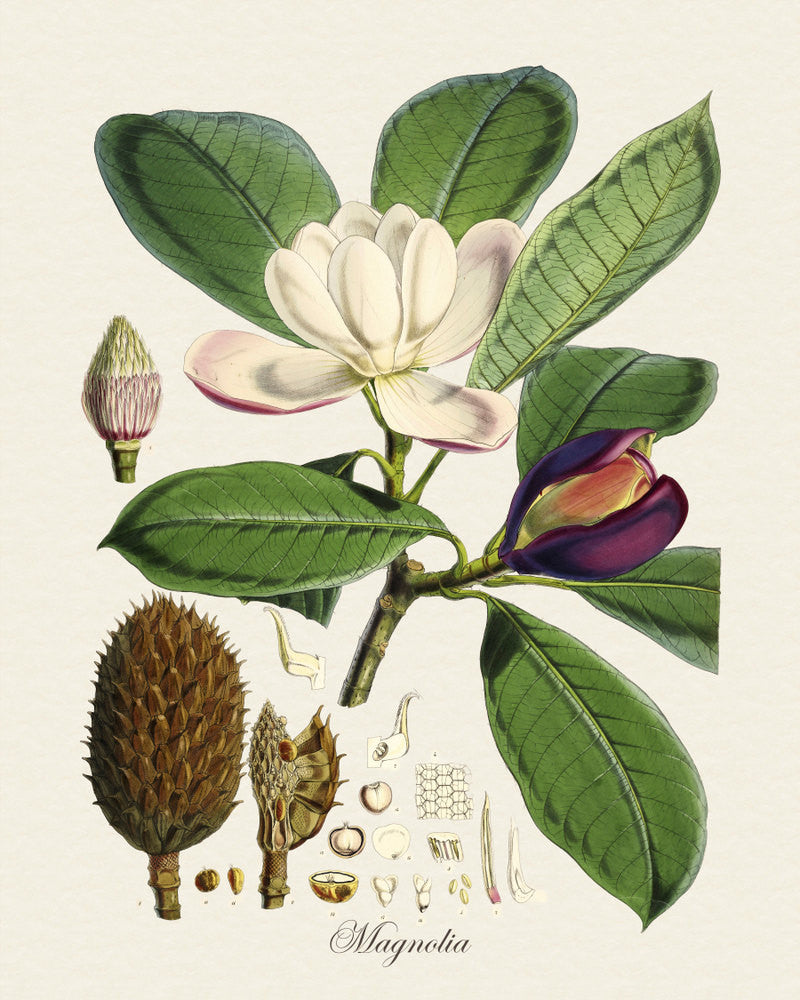This rectangular, portrait-oriented drawing showcases a beautifully detailed magnolia flower in the center, partially open with its delicate white petals unfurling gracefully. Below the flower, "Magnolia" is elegantly inscribed in black cursive font. To the right of the main bloom, a flower bud encased in a dark purple shell stands poised to blossom. Surrounding the flowers, large, cylindrical green leaves form a lush backdrop. On the left side, another plant with a cylindrical shape and a pointed top adds contrast to the composition. The base of the drawing is adorned with an assortment of additional plants in hues of brown, white, and yellow, all contributing to the rich botanical tapestry.